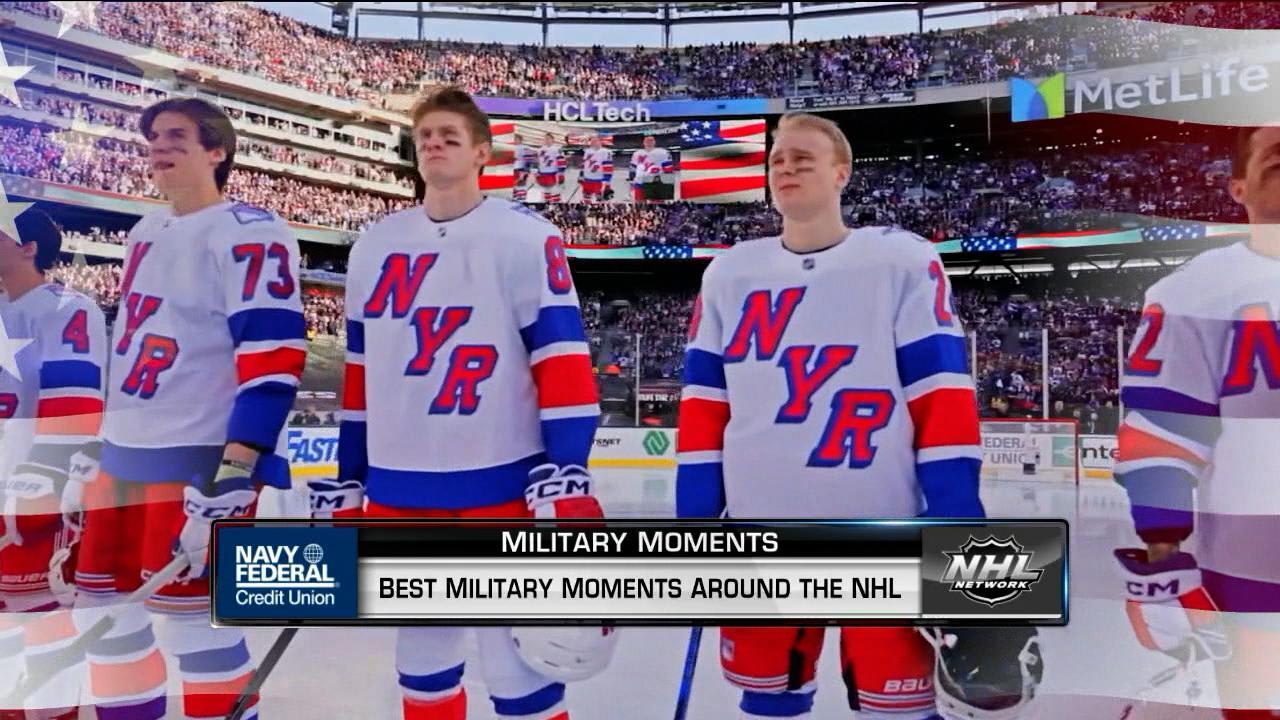In the image, a landscape-oriented screenshot from a hockey video game, we see five white male players lined up on the ice, all facing forward and holding their helmets. They each wear white jerseys with long sleeves that feature blue, red, and blue stripes, and prominently display "NYR" in bold red letters with a blue border. Below the players, there's a banner that says "Military Moments" in white text on a black bar, with "Best Military Moments Around the NHL" written in black text inverted on a white bar beneath it. On the left of the banner is a Navy Federal Credit Union logo, while the right side bears the NHL Network logo. The background reveals fully packed stands, and the quality of the image is notably blurry, reinforcing its video game-like appearance.